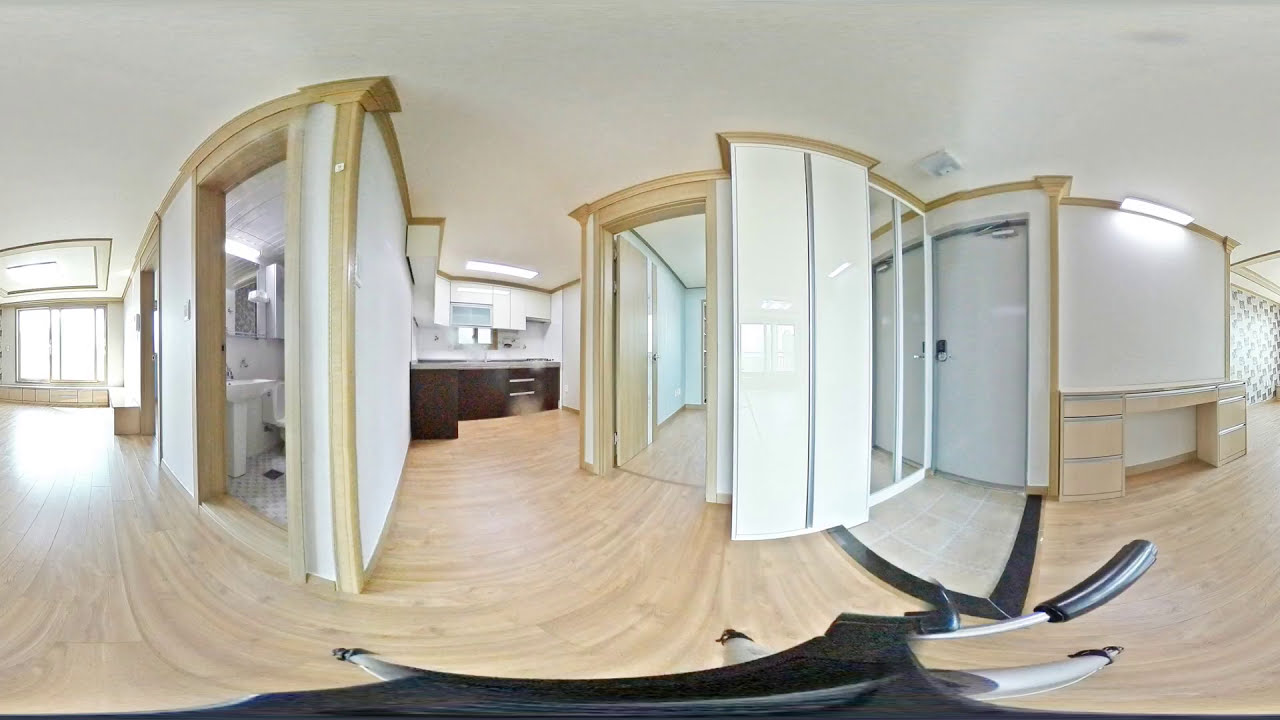This image appears to be a distorted, fisheye-lensed photograph of an unfurnished apartment interior, creating a panoramic and somewhat disorienting view. The apartment features light tan wooden floors, white walls, and a white ceiling. The flooring has a swirling pattern due to the lens distortion, emphasizing the fisheye effect. On the left side of the photograph, there are large windows allowing ample natural light into the space. The central part of the image showcases the kitchen, equipped with modern dark brown or black lower cabinets, contrasting white upper cabinets, and white countertops. To the right, there appears to be a bathroom with white fixtures, including a visible sink and toilet, and beige diamond-patterned floor tiles. Adjacent to the bathroom, there's a closet or bedroom with light wooden drawers and space potentially for a TV, marked by sliding white doors. The overall color palette is neutral, featuring shades of black, white, gray, silver, dark brown, and light brown, with no visible text or additional decorative elements, highlighting the apartment's modern yet empty state.